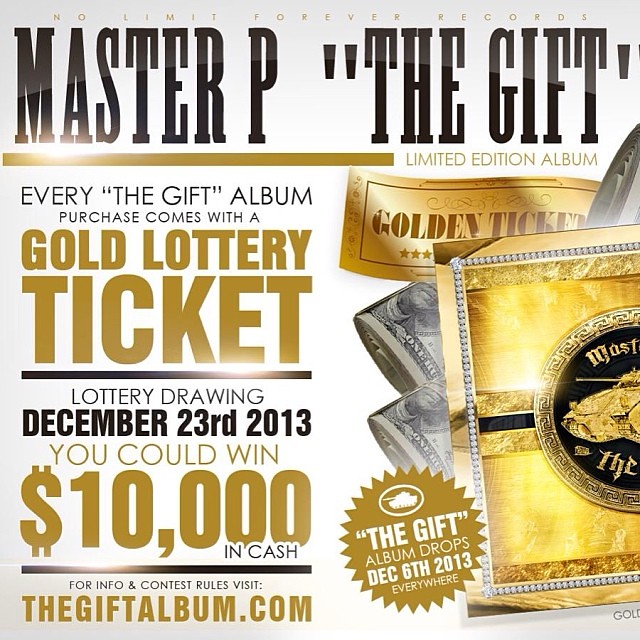This advertisement for No Limit Forever Records showcases Master P's limited edition album, "The Gift." The detailed image features a clean white background with intricate black and gold elements. The top of the advertisement displays the No Limit Forever logo in small gold lettering, while prominently underneath in black ink, it reads "Master P The Gift Limited Edition Album." Scattered around the ad, there are three wadded rolls of $100 bills, adding a luxurious touch.

Central to the design are multiple gold tickets, with one prominently labeled "Golden Ticket," and another featuring a golden tank, symbolizing Master P’s brand. One of these tickets, partially cut off, shows the words "Master" at the top and "The Gift" at the bottom, reinforcing the album’s title.

A significant promotional detail is highlighted on the left side: "Every 'The Gift' album purchase comes with a gold lottery ticket." Below this, it notes that the lottery drawing will be held on December 23rd, 2013, with a chance to win $10,000 in cash. The album will be available everywhere starting December 6th, 2013. Prospective buyers are directed to visit TheGiftAlbum.com for more information and contest rules. This extensive information is elegantly presented in a mix of black and gold lettering.